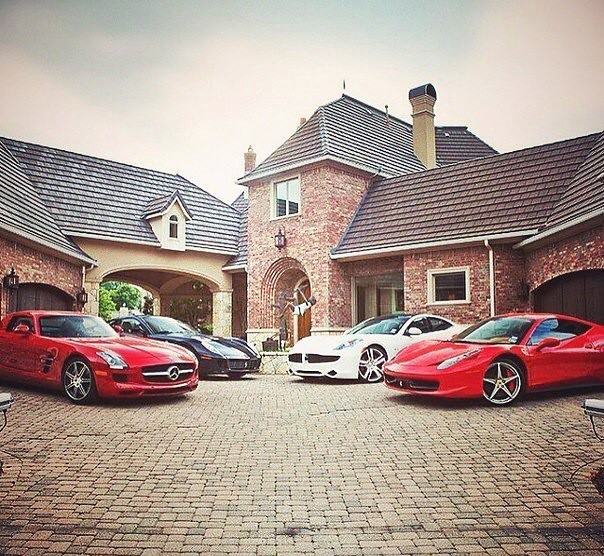The image captures a lavish display of automotive opulence, featuring four flashy sports cars parked on a light grey cobblestone driveway in front of an expansive red brick house with a sloping gray-black tiled roof and a white chimney. The two red sports cars are situated at the front, flaunting their sleek roofs, while a black sports car and a white sports car are positioned diagonally behind them. The grand residence boasts a prominent entrance with a large archway, a statue, several windows, and just the edge of a dark wood-paneled garage door. To the left, a white stucco connecter with a drive-through overhang leads to another red brick section of the house. The entire scene seems designed to showcase the homeowner's impressive collection of luxury cars in front of their elegant home.